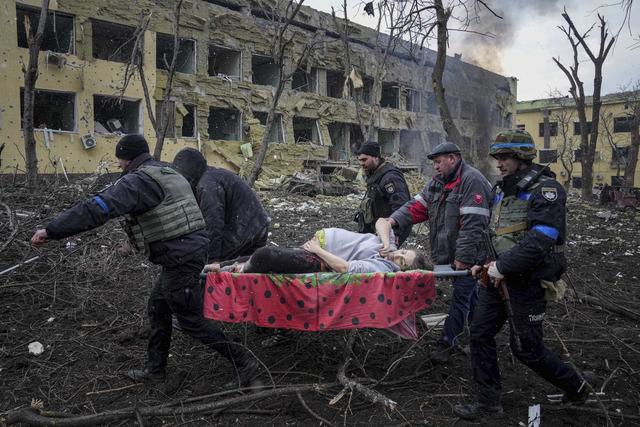In this evocative outdoor image, the harrowing aftermath of conflict is evident. At the heart of the scene is a dilapidated and decrepit apartment building in the background, heavily marred by bullet holes and bomb damage, with a greenish-yellow tint, indicative of fire damage and neglect. Thick smoke lingers in the air, adding to the desolate ambiance. The building’s windows are blown out, and the surrounding trees appear charred and leafless, further emphasizing the devastation.

In the foreground, chaos and urgency are palpable as five men, seemingly of Ukrainian affiliation due to the blue ribbon straps on their sleeves, hastily transport a woman on a stretcher. The men are clad in dark clothing, including dark coats and a noticeable dark green vest. One of them, distinguished by a helmet, appears to be a soldier, contrasting with the others who wear various hats. Amidst the scattered debris and the cold weather indicated by everyone’s warm attire, a figure of a fire professional with a helmet adds to the scene’s complexity and sense of emergency.

This poignant image not only captures the immediate response to a catastrophic fire and possibly battle, underscoring the profound human impact and desperation in a war-torn setting.